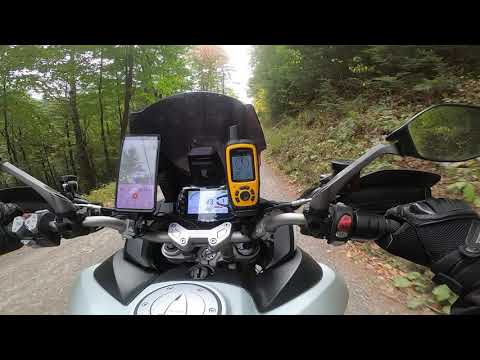Captured from the rider's perspective, the image centers on a silver motorcycle featuring black accents and a black-tinted visor. The rider's gloved hands, prominently visible, grip the handlebars, with the right hand mostly shown. Both handlebars are equipped with mirrors, while the middle section holds multiple technology devices — including a GPS screen and two cell phones, one of which is yellow. The scenery around reveals a narrow path winding through a dense forest area, flanked by trees laden with leaves. A bright white sky filters through the foliage on the left side, accentuating the natural setting. The photo seems to have been taken with a device like a GoPro, emphasizing the immersive and dynamic viewpoint of a ride through the woods on a sunny day.